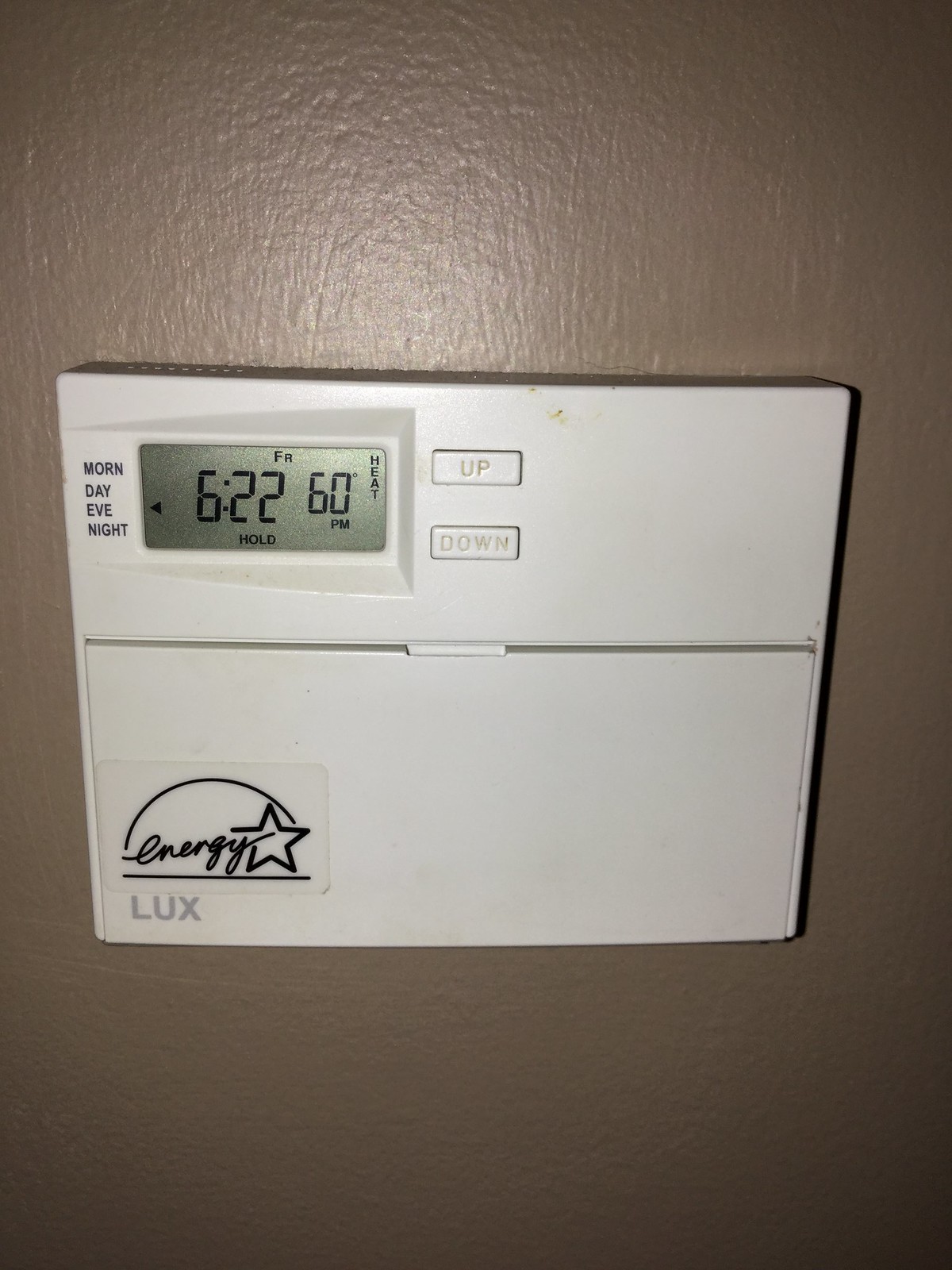A white, squarish LUX thermostat with rounded corners is mounted on a gray wall with a warm amber undertone. The thermostat's screen displays "622" and "hold," indicating that the device is set to 6:22 PM and is currently in heating mode. An arrow on the screen points towards the evening setting. The thermostat features up and down buttons for adjusting the temperature.